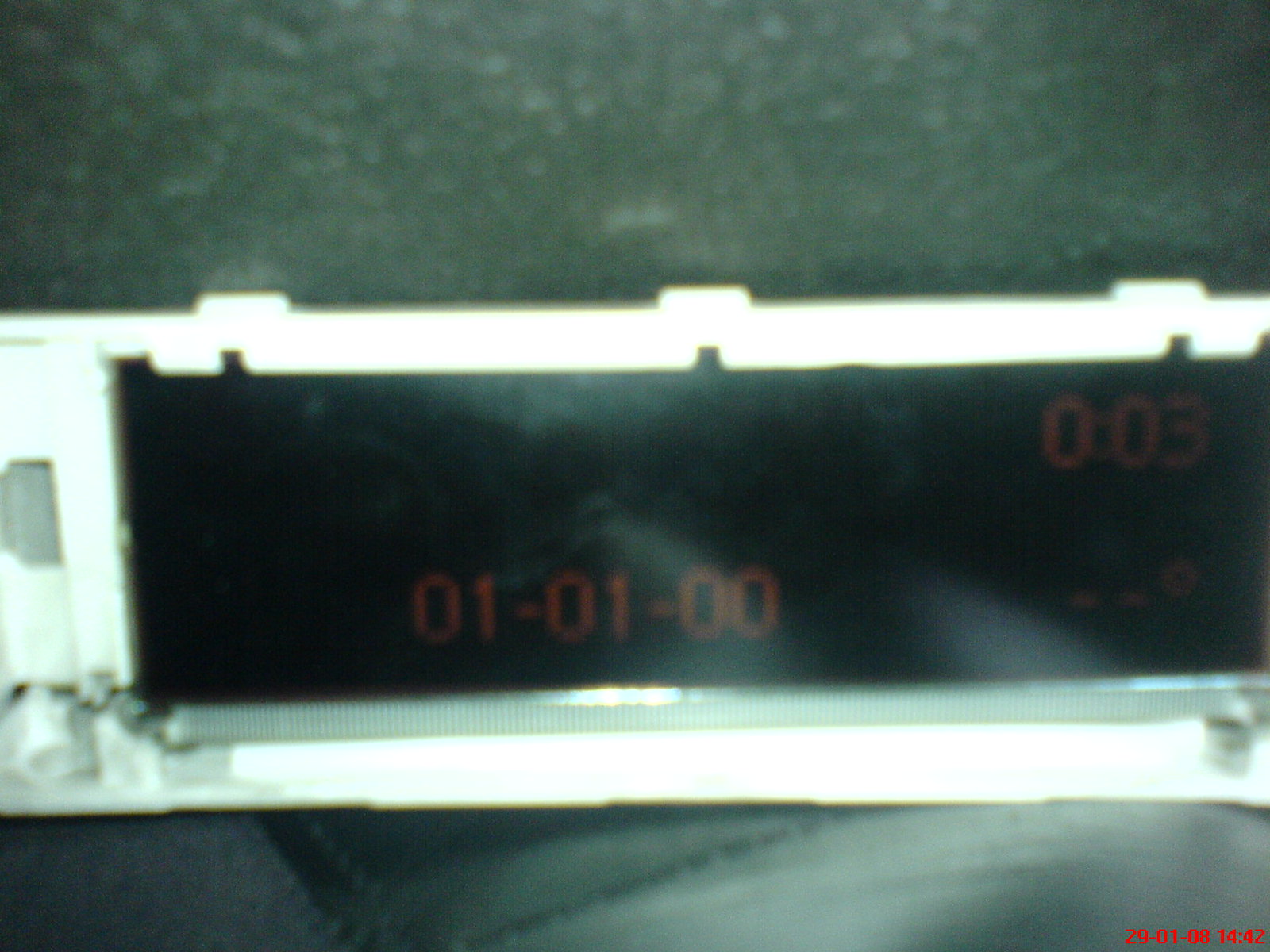The photo captures a rectangular, silvery-white metallic device placed centrally on a textured gray surface. The surface features a leather-like grain in the top half, transitioning to a smoother texture beneath. The image appears slightly blurry and out of focus. The device has a black screen in its center, which displays multiple pieces of information. In the middle-bottom of the screen, it reads "01-01-00" in red text. In the top-right corner, "003" is displayed in the same red lettering. Close by, it shows two dashed marks followed by a temperature symbol, although no specific temperature is visible. The bottom right-hand corner of the photo contains the date and time: "29-01-08 14:42" in red text. Additionally, there's detailing on the left side of the device, possibly for a screw. The textured gray background likely consists of a black granite-like material with white dots, resembling a countertop, complemented by a leather-like bottom section.